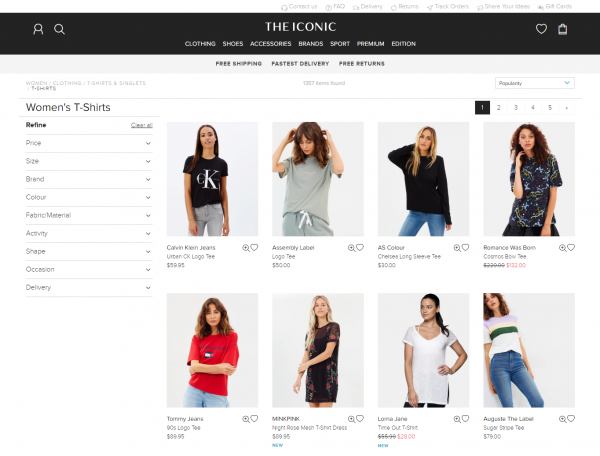Screenshot of The Iconic's Website: 

At the top of the website, a sleek black banner features the logo "The Iconic" at its center, flanked by category links including Clothing, Shoes, Brand, Sport, Premium, and Edition. To the right, additional hyperlinks offer navigation to pages like Contact Us, FAQ, Delivery, Returns, Track Order, Share Your Ideas, and Gift Cards. Iconic utility logos such as hearts, a search function, a user profile, and an external link are also situated on this black banner.

Below this, a gray banner highlights service perks with text proclaiming Free Shipping, Fastest Delivery, and Free Returns.

Towards the bottom right of the screen is a collection of eight images showcasing women modeling various t-shirts. The lineup includes a black Calvin Klein tee, a gray large-logo t-shirt, a black long-sleeve shirt, another black patterned t-shirt, a white tee with stripes in purple, yellow, and green, a casual white long v-neck t-shirt, a t-shirt dress, and a red shirt emblazoned with "Tommy Jeans." Each item features its price with a magnification option for closer viewing.

On the bottom left side, a section titled Women's T-shirts offers filters to sort the products by attributes like price, size, brand, color, fabric material, activity, shape, occasion, and delivery options.